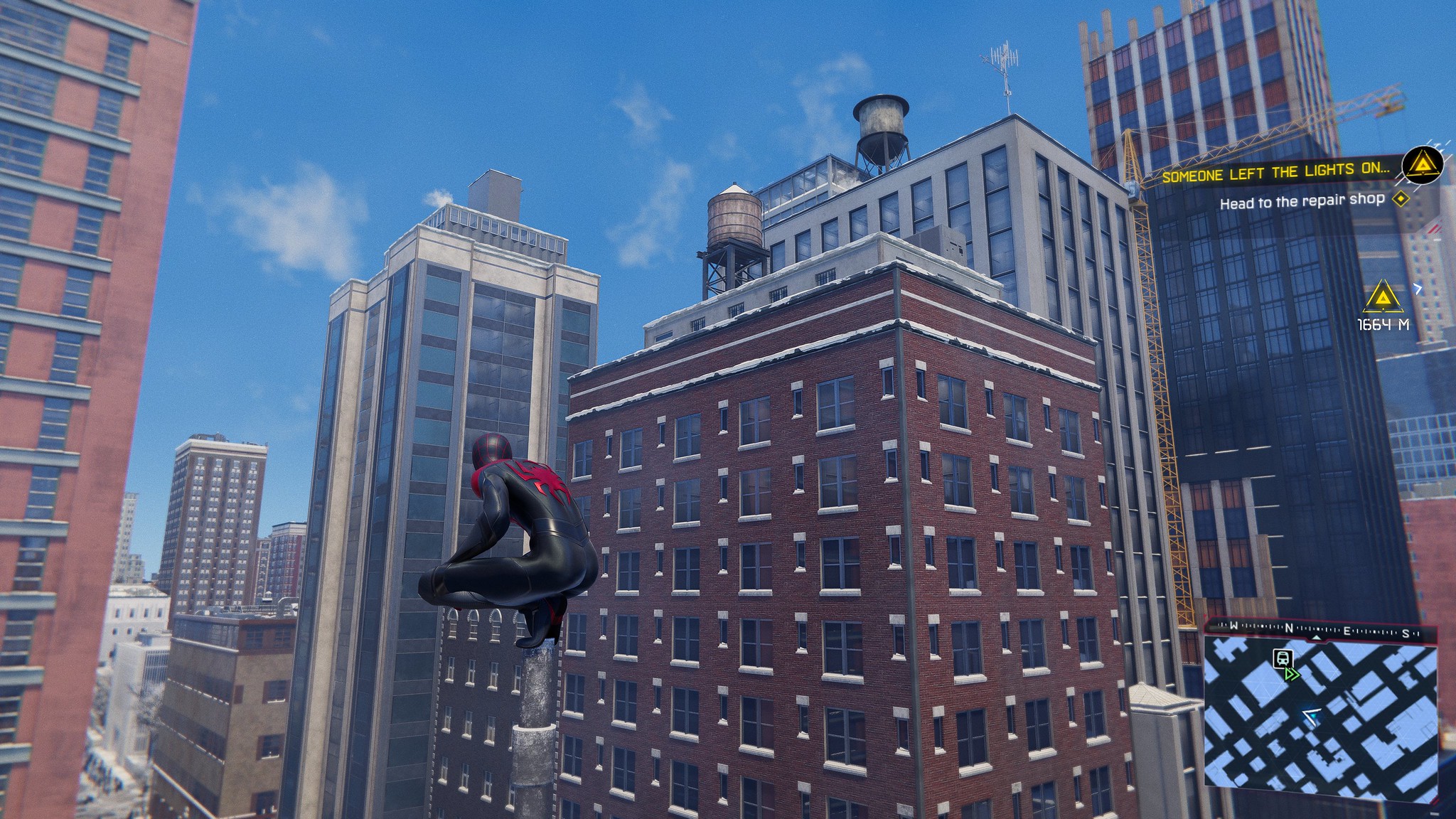This image is a screenshot from a Spider-Man video game, potentially titled "No Way Home." Dominating the center of the picture is Spider-Man, donned in his distinctive black suit with the striking red spider emblem. He is poised in his iconic crouch atop a very small antenna-like structure, exuding readiness and agility. Surrounding him are the urban elements of the cityscape, with various buildings featuring architectural details like water towers perched on their rooftops. 

On the right side of the screen, a mission prompt in yellow text reads, "Someone left the lights on. Head to the repair shop," followed by a distance indicator showing "1664 meters." At the very bottom of the image is a map interface, providing directional guidance for the player. The scene is set during daytime, evident from the blue sky adorned with soft, billowy, and wispy clouds, adding a serene backdrop to the bustling city environment.